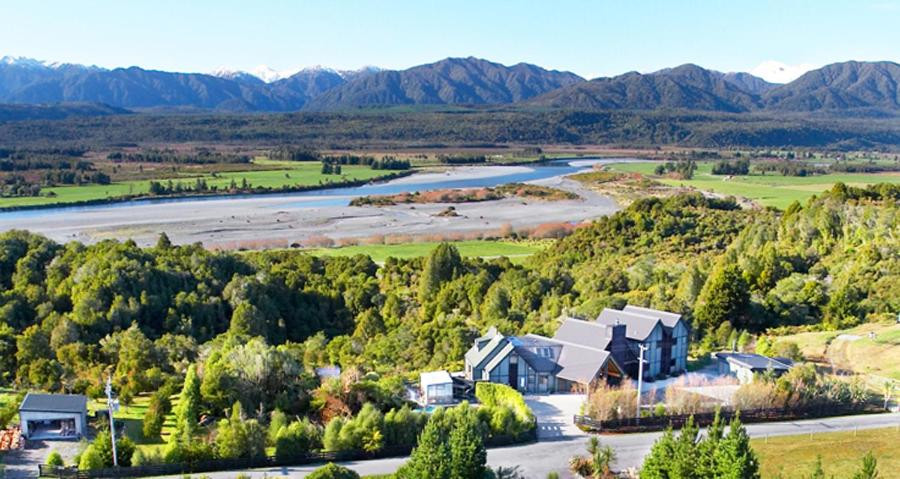This detailed aerial image showcases the breathtaking landscape of Hokitika, New Zealand, centering on the Raimu Lodge located on the South Island. Dominating the lower portion of the image is a long, gray road cutting across the frame, providing access to a grand, mansion-style lodge that features distinct alpine architectural elements, including steep roofs and visible cross members. The lodge stands out with its multiple buildings, painted in a sophisticated palette of white and gray.

In front of the lodge, an expansive green lawn stretches out, hinting that this property might be isolated without much neighboring residential development. Behind the lodge, a dense sequence of woodland trees offers a natural barrier, transitioning seamlessly into a leveled area of varied vegetation that further merges into sandy banks bordering a serene blue river. This river reflects the vivid blue sky above, which is so bright that it appears almost white near the horizon.

Beyond the river, more forested regions span out, leading up to a dramatic series of mountain ranges in the background. These mountains display shades of green and brown, with the most distant peaks adorned with snow caps, adding to the picturesque alpine atmosphere. The vibrant greenery, alongside dense forests, sunny patches, and water elements, all come together to create a harmonious and diverse landscape, encapsulating the beauty and tranquility of rural Hokitika, with the Raimu Lodge as its architectural jewel.